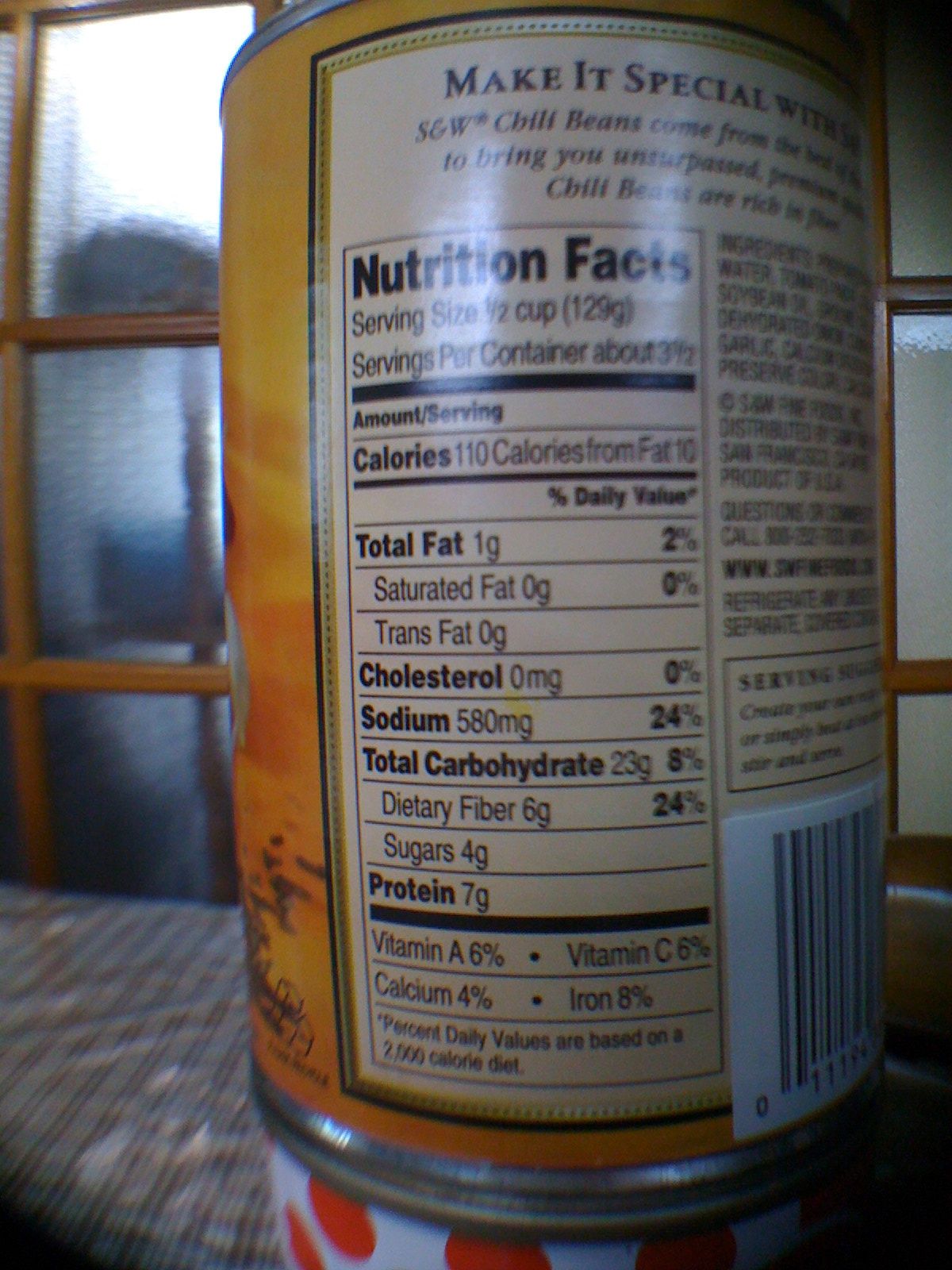This vibrant color photograph provides a close-up view of the back of a can of food, highlighting its nutritional information. The left side of the image reveals a portion of the can's label, which features a striking blend of orange and yellow shades. Dominating the center of the image is the "Nutrition Facts" section, clearly displayed. Above this nutritional information, a partly blurred headline reads "Make It Special," followed by the more legible "Chili Beans," hinting at the can's contents. The nutritional summary indicates that a half-cup serving of these beans contains 110 calories, 10 grams of fat, 580 milligrams of sodium, 23 grams of carbohydrates, 6 grams of dietary fiber, 4 grams of sugar, and 7 grams of protein. Additionally, the lower right-hand corner of the can features a distinct barcode, completing the detailed view of this everyday kitchen staple.